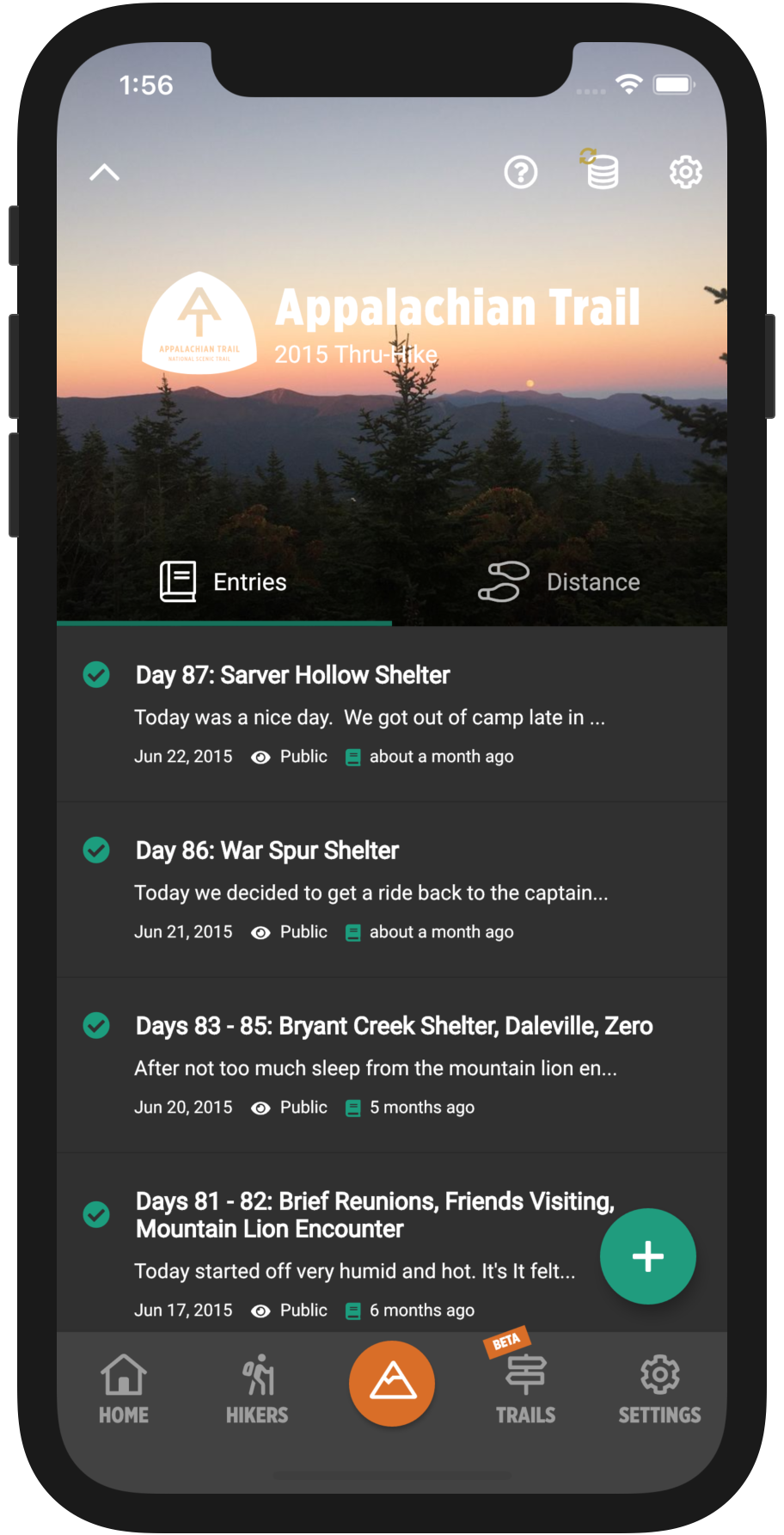The image depicts a close-up of a smartphone screen, which appears to be an iPhone, as suggested by the user interface design. The top left corner of the screen shows the time as 1:56, while the top right corner indicates that the device is connected to Wi-Fi and has a full battery charge. The screen displays an app that seems to cater to hikers, specifically those trekking the Appalachian Trail.

At the top of the app, "Appalachian Trail" and "2015 Thru Hike" are prominently featured. The user has selected the "Entries" tab, which is marked with a book or journal icon, next to the "Distance" tab, identified by an icon of two footsteps. 

The first entry under the "Entries" tab is titled "Day 87: Sarver Hollow Shelter." It starts with, "Today was a nice day. We got up camp late in..." followed by an ellipsis, indicating more content that can be viewed by tapping on it. This entry was posted on June 22, 2015, made public, and was uploaded about a month ago. 

The second entry, "Day 86: Four Pines Hostel," begins with, "Today we decided to get a ride back to the captain's cabin..." and also ends with an ellipsis. It was posted on June 21, 2015, made public, and uploaded about a month ago. 

Another notable entry titled "Days 83-85: Bryant Ridge Shelter to Daleville" mentions, "Zero after not much sleep from the mountain lion..." with an ellipsis indicating more content. Dated June 20, 2015, it was made public about five months ago. 

The entry for "Days 81-82: Reunions with Friends; Mountain Lion Encounter" starts with, "Today started off very hot and humid..." and is also truncated with an ellipsis. This was posted on June 17, 2015, marked public, and uploaded six months ago.

At the bottom of the app, several tabs are visible: "Home," denoted by an icon resembling a house, "Hikers," "Trails," marked with a "beta" tag, and "Settings." This neatly organized interface suggests comprehensive features aimed at helping hikers track and journal their journey on the Appalachian Trail.